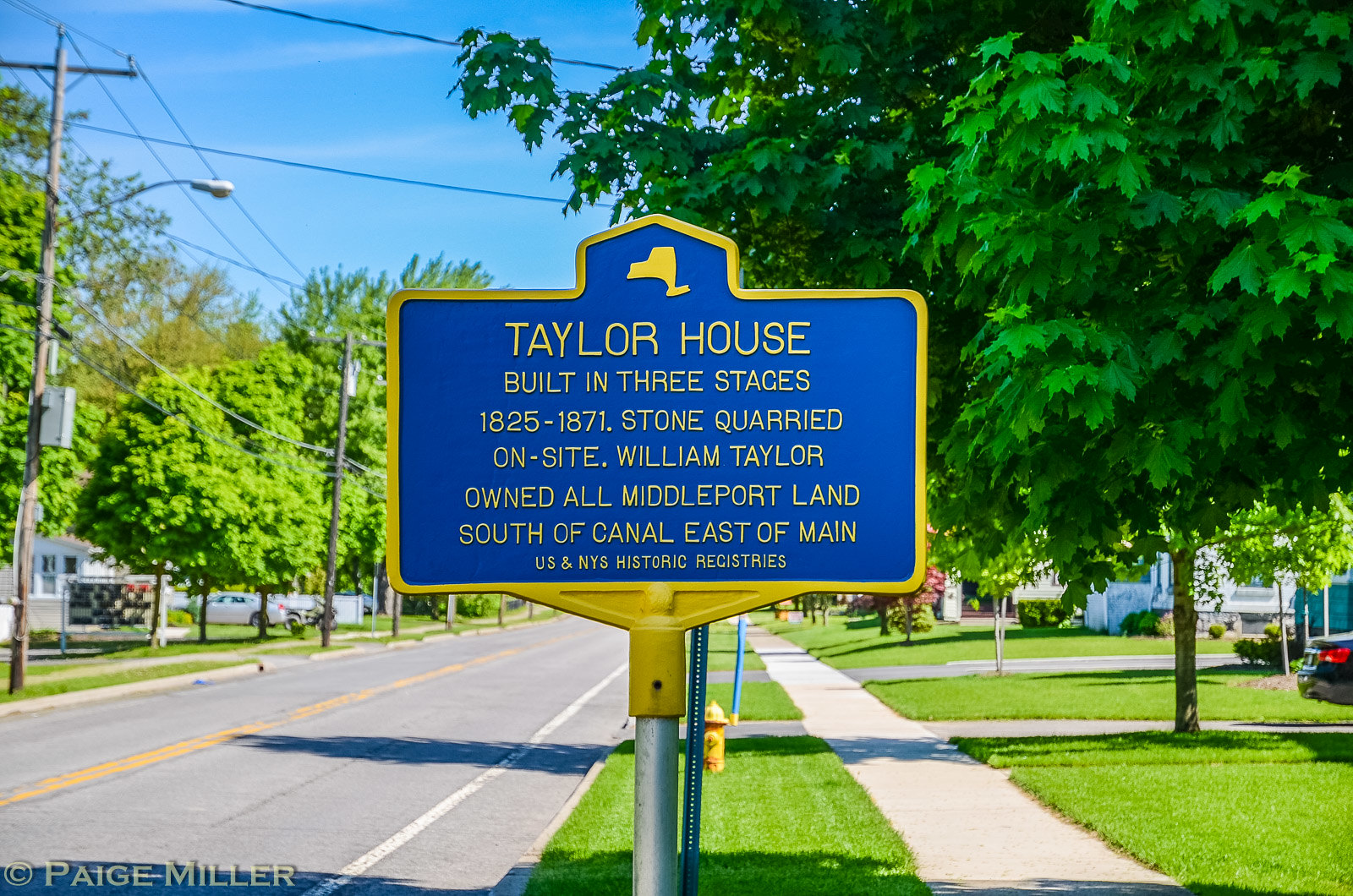This wide, rectangular image captures a historical marker along a quiet street in a well-kept, middle American town on a bright summer day. The sign, mounted on a silver pole, is dark blue with yellow borders and text, featuring a small house-like shape at the top. It reads in all capital letters: "TAYLOR HOUSE built in three stages, 1825 to 1871 stone quarried on site. William Taylor owned all Middleport land south of Canal, east of Maine.” 

To the left of the sign, a gray paved road with two yellow stripes down the middle and a white stripe at the edge runs into the horizon, disappearing behind the sign. The road is empty at the moment. To the right, a narrow, light gray sidewalk also stretches into the distance, bordered by well-maintained bright green lawns. These lawns are dotted with tall, vivid green trees, their tops cut off by the image's frame. In the distance, a black car is parked near a driveway, complementing the serene suburban atmosphere. The sky above is a bright blue, indicating a clear, sunny day, enhancing the vibrant colors and the overall tranquil feel of this typical American town scene.